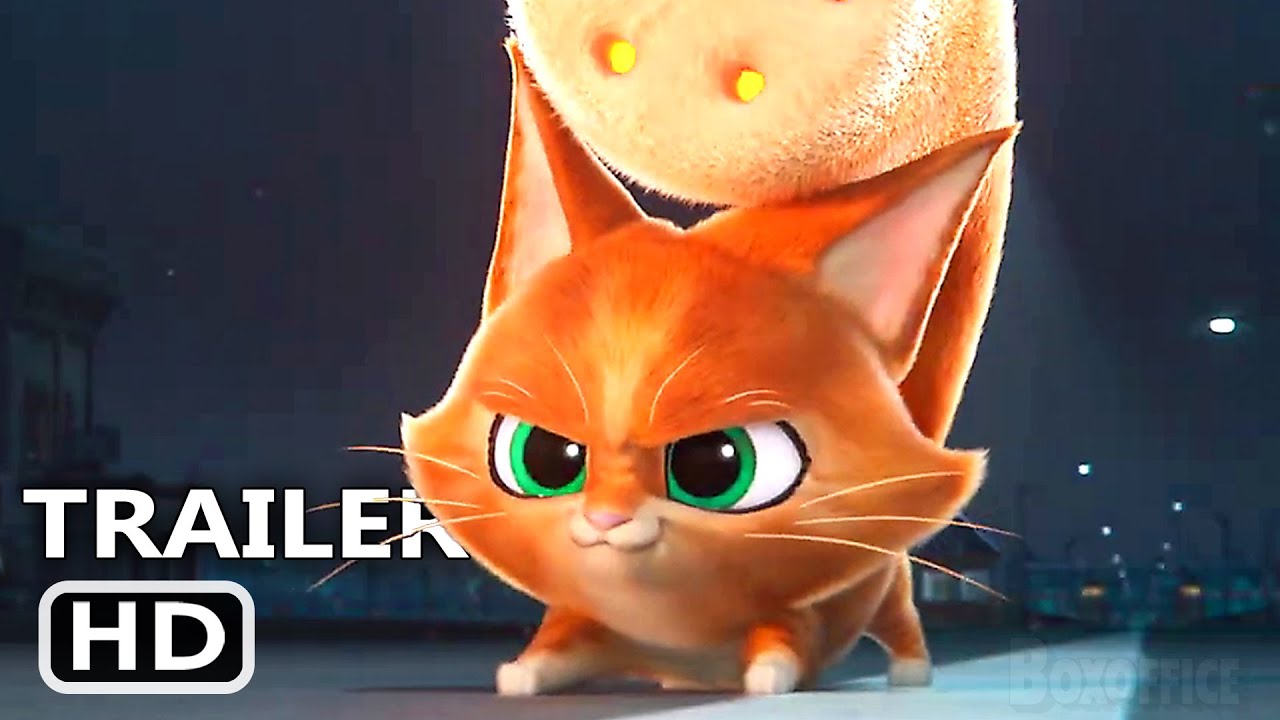In this detailed image from the 2022 animated movie "DC League of Super Pets" trailer, a squat orange cat with pointed ears and intense green eyes is the focal point. The cat, depicted as a cartoon character, has a serious scowl, with little whiskers on its face. Its disproportionally large head and extremely short legs make its tummy appear to be dragging on the ground. The cat's tail, rising behind it on the right, features holes through which yellow light shines, resembling whiskers and adding an odd, whimsical touch to its otherwise serious demeanor. The dark background subtly reveals some lights, buildings, and sky, enhancing the dramatic tone of the scene. The bottom left corner of the image is marked with the text "trailer HD," indicating its source from the movie trailer. This striking and curious image effectively represents the "DC League of Super Pets" animated film.